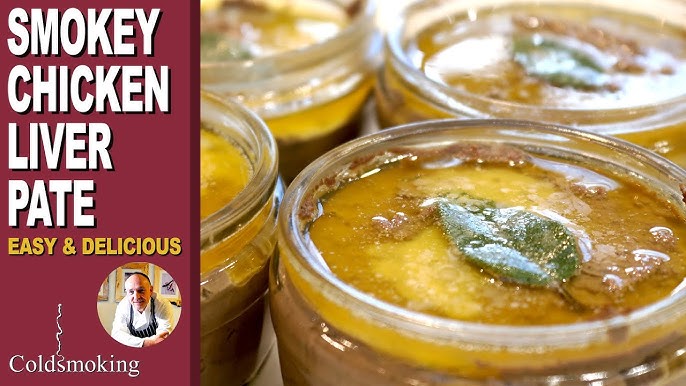This image appears to be an advertisement for "Smoky Chicken Liver Pâté." The left side features a dark reddish-purple vertical stripe extending halfway across the horizontal rectangle. In white text, outlined in black, it says "Smoky Chicken Liver Pâté," and in gold, "Easy and Delicious." Below, in white text, it reads "Cold Smoking." Also on the left, within a circle, there's a photo of an elderly bald man, likely in his 70s or 80s, smiling into the camera. He is wearing a white collared long-sleeve shirt and a blue or black apron, with his arms crossed over his chest. Behind him are wooden-framed images or decorations.

On the right side of the advertisement, there are close-ups of open glass mason jars filled with a golden mustard-brownish substance, presumably the pâté. Each jar is crowned with a green leaf on top. The forefront is in focus, showcasing the vibrant colors and texture of the contents, while the background is slightly blurred. The lighting in the image enhances the visual appeal, suggesting professional or semi-professional photography. This detailed presentation combines to effectively promote the artisanal and appetizing qualities of the chicken liver pâté.